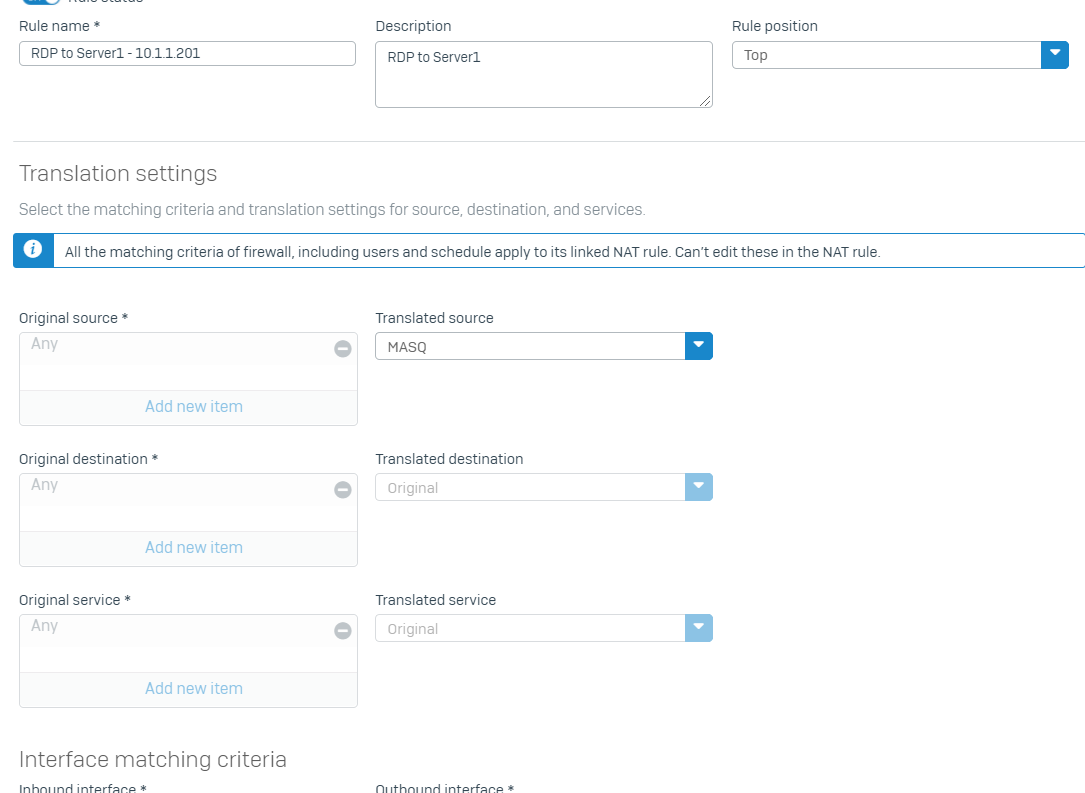The image depicts a section of a website focused on translation settings and firewall configurations. The main header of the section is partially cut off, but it is evident that the page deals with network and firewall settings. The main content area consists of several sections:

1. **Translation Settings**: A directive to select the matching criteria and translation settings for various elements such as the source, destination, and service. 

2. **Firewall Matching Criteria**: A note indicating that the matching criteria for the firewall, which includes users and schedules, apply to the link. Additionally, NAT (Network Address Translation) rules can be edited here.

3. **Criteria Details**:
   - **Original Source**: 'Any'
   - **Original Destination**: 'Any'
   - **Original Service**: 'Any'

   There are options to add new items for these criteria, but currently, no additional items have been added.

4. **Interface Matching Criteria**: Though the section on interface matching criteria is truncated, it includes:
   - **Translate Source**: Set to 'M-A-S-Q', with a dropdown menu for further modification
   - **Translate Destination**: Set to 'Original', with a dropdown menu
   - **Translate Services**: Set to 'Original', with a dropdown menu
   - **Outbound Interface**: Information partially cut off

The entire section is laid out against a white background, and the website uses a color scheme of white, black, gray, and various shades of blue, adding a subtle color gradient from darker blue to lighter blue. The overall design appears to be clean but is somewhat obscure due to the cutoff in the upper section.